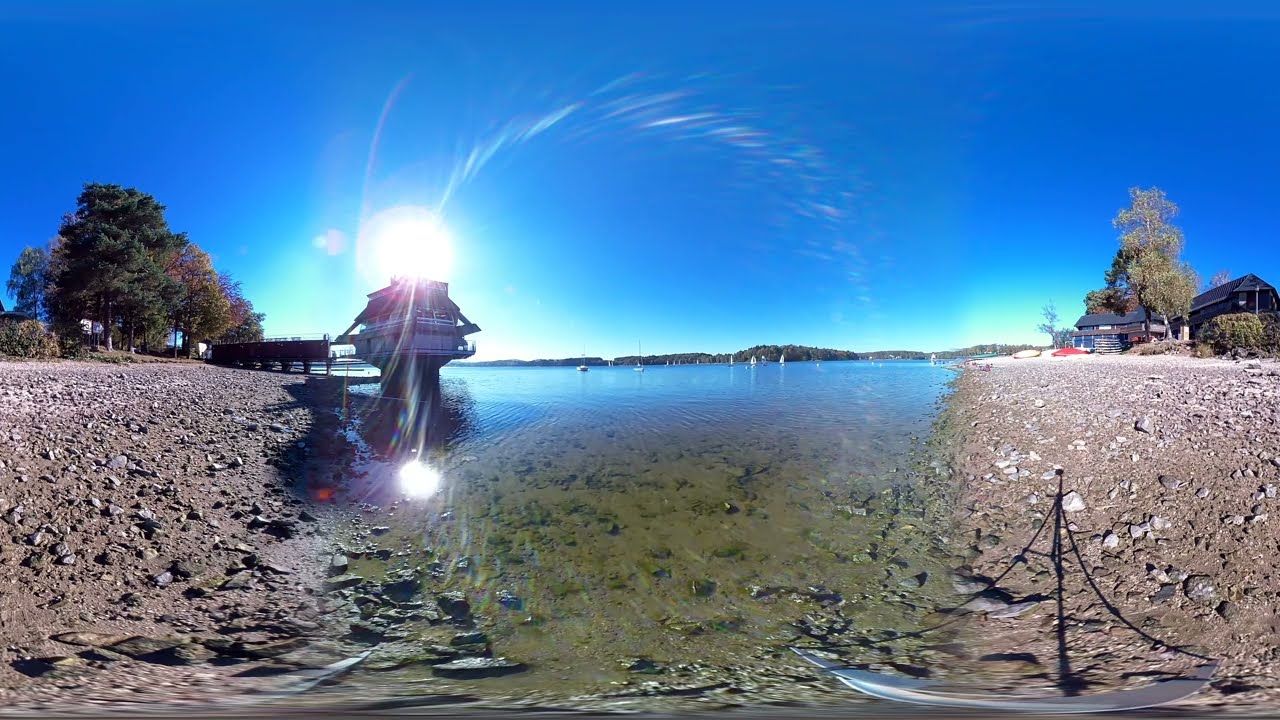This panoramic image captures a stunning lakeside scene bathed in clear, late afternoon sunlight. The sky is an impeccable, cloudless blue, creating a beautiful contrast against the greenery of large trees scattered along the shoreline. The calm, mirror-like water reflects the scenery perfectly, transitioning from an algae-green near the shore to a deeper blue further out.

On the right side of the image, a house nestles close to the rocky shore, partially obscured by a large tree in front. A red kayak rests nearby, emphasizing the tranquil, recreational vibe of the scene. In the middle of the image, the lake stretches out, hints of boats visible against a backdrop of verdant mountains, enhancing the sense of depth and natural beauty.

Towards the left, a dock extends out to a structure built over the water, resembling a house on a platform, connected to the shore by a bridge. The sun is low, creating a lens flare effect above this building, adding warmth and capturing the serene, end-of-day ambiance. The gravelly, rocky shore continues beneath the water's surface, visible through the crystal-clear, undisturbed lake.

Overall, the image epitomizes a serene and picturesque lakeside retreat, with the natural beauty complemented by the human-made structures harmoniously blending into the landscape.